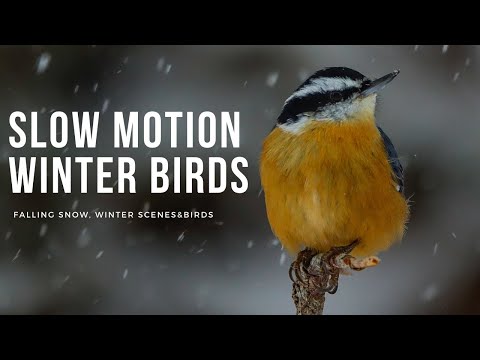The image features a small bird perched on a tiny branch on the right side. The bird has an orange chest, a black and white striped head with a sharp, medium-length black beak, and part of its black wing is visible near the right side of its body, which also has some brown feathers. The bird's head is tilted to the right. The background is a blend of gray, white, and black, with snow falling, creating a wintry atmosphere. The background appears out of focus, emphasizing the bird in the foreground. On the left side of the image, large white capital letters read "SLOW MOTION WINTER BIRDS" with smaller white text below stating "falling snow, winter scenes, and birds." The overall scene appears to capture a serene winter day, highlighting the bird in its natural habitat.